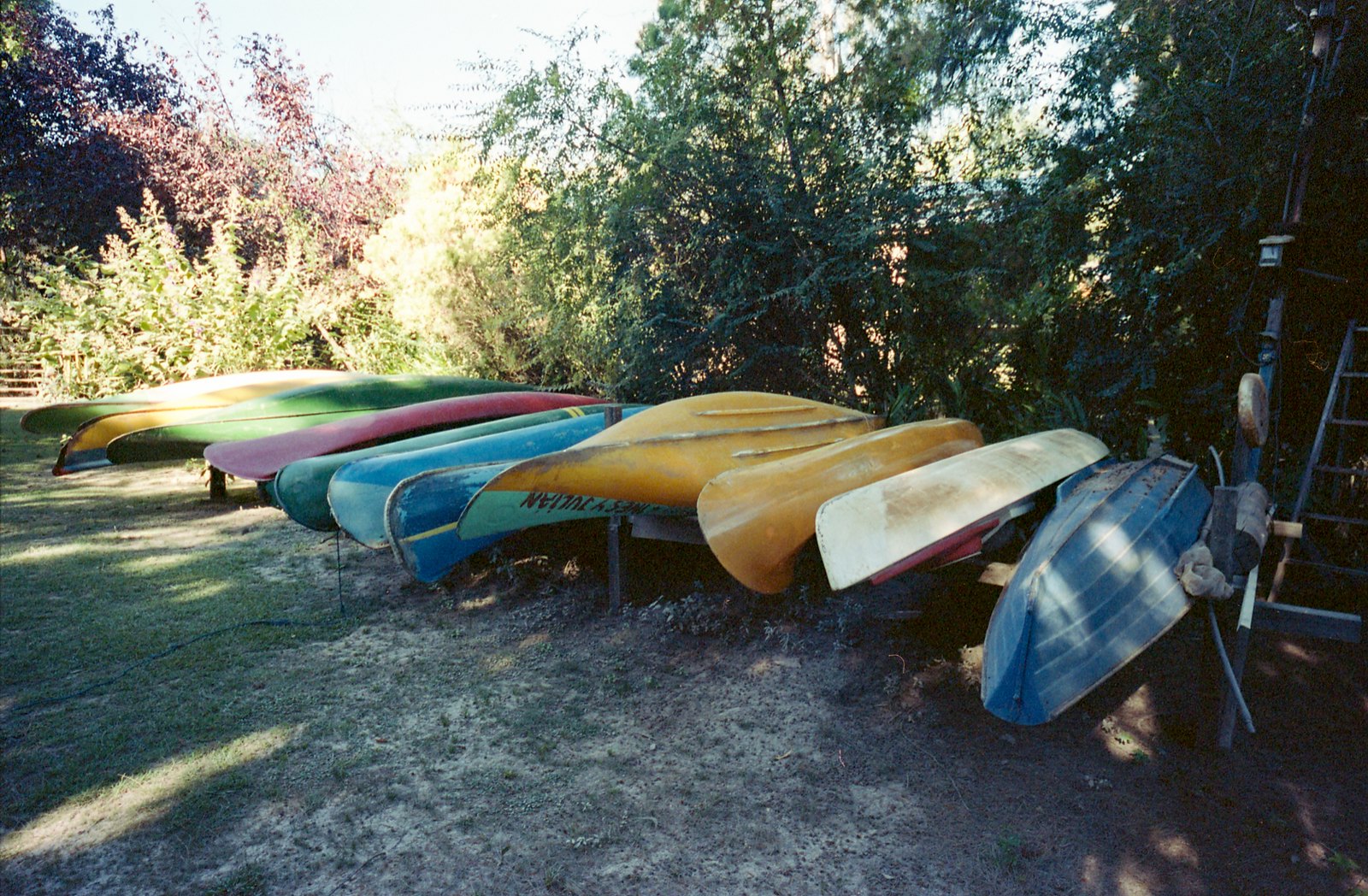This color photograph captures a scene likely near a lake or stream, featuring a patchy grassy area with dirt and partial sunlight filtering through the trees. A line of canoes is prominently displayed in the foreground, positioned on metal brackets off the ground, drying with their backs up and seats facing down. The canoes proceed from right to left, showcasing a diverse array of colors in the following order: blue, white, two yellows (the second yellow featuring a navy blue mast), light blue, green, red, two more blues, another green, yellow, and finally, another green. The background reveals a blend of trees, bushes, and hedges, with a partly overcast sky visible above. At the far right of the image, some oars are noticeable, and a ladder is propped against an unseen structure, adding to the sense of an organized, possibly rental, canoe storage area.